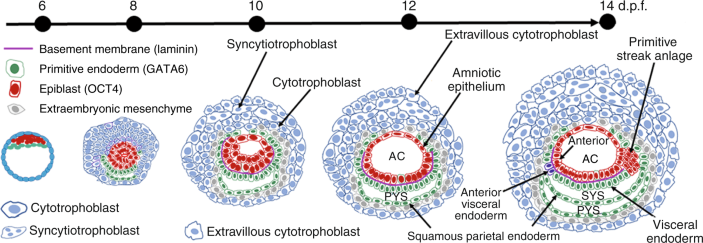This horizontal image with a white background is a detailed scientific diagram illustrating the differentiation and growth of early human embryos from day 6 through day 14 post-fertilization (DPF). Starting on the left, the sequence begins with a small blue cell and progresses through five stages of increasing size toward the right. Each stage is depicted with a blue outer layer (cytotrophoblast), a red interior region (epiblast), and green lines (primitive endoderm). 

The diagram includes a timeline at the top labeled with days post-fertilization (6, 8, 10, 12, 14), with specific points corresponding to each illustrated stage. A key or legend explains the color coding and various parts of the growing cell: purple lines indicate the basement membrane, green lines denote the primitive endoderm, red represents the epiblast, and gray shows the extraembryonic mesenchyme. Blue markings indicate cytotrophoblast, with blue squiggles representing syncytiotrophoblast. 

In more detail:
- At day 6, the blue cytotrophoblast forms the exterior layer, encapsulating the red epiblast and green primitive endoderm.
- By day 8, the epiblast begins to grow, and the diagram shows further differentiation.
- At day 10, the cytotrophoblast begins expanding into syncytiotrophoblast as the epiblast continues to fill the cell.
- At day 12, the primitive endoderm and extraembryonic mesenchyme develop, and the amniotic epithelium starts taking shape within the epiblast.
- By day 14, the epiblast and primitive endoderm separate further, forming a central amniotic space and initiating the appearance of the primitive streak.

The intricate layers and components, like the anterior visceral endoderm and squamous parietal endoderm, are also indicated, showcasing the complexity of early embryonic development. Each stage visually explains how different types of cells such as extravillous cytotrophoblast evolve and structurally contribute to the embryo's growth.